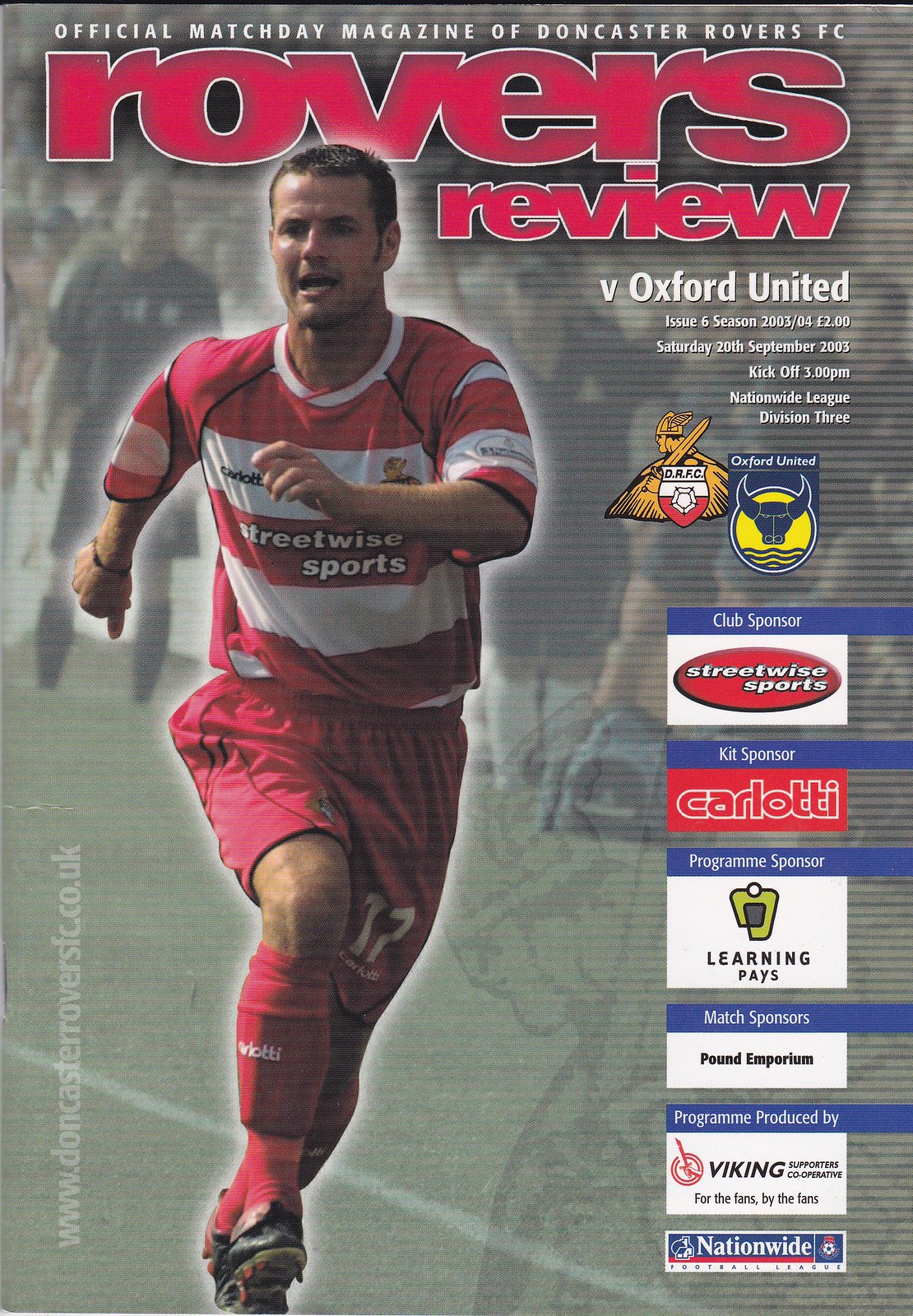The cover of the magazine, titled "Rovers Review," showcases a dynamic image of a soccer player in his late 20s or early 30s, sprinting on the field. He is donned in the red and white kit of Doncaster Rovers FC, featuring a striped shirt with the sponsor, Streetwise Sports, emblazoned in white, red shorts, and red socks over shin pads, paired with black cleats. The background subtly captures spectators on the sidelines and in the stands, adding to the vibrant matchday atmosphere.

At the top of the cover, the magazine declares itself as the "Official Match Day Magazine of Doncaster Rovers FC," with further details indicating it is Issue 6 of the Season 2003-04. The match is against Oxford United, scheduled for Saturday, 20 September 2003, at 3 p.m., as part of the Nationwide League Division III. The cover price is marked at £2.

Notably, several logos adorn the cover, including those of DRFC, depicted as a Viking with wings and a shield, and Oxford United, represented by a blue bull's head on a yellow circle with water lines at the bottom. Sponsorship information is prominently displayed: Club Sponsor, Streetwise Sports, Kit Sponsor, Carlotti, Program Sponsor, Learning Pays, and Match Sponsor, Pound Emporium. The program is produced by the Viking Supporters Cooperative, for the fans by the fans. The cover also directs readers to the club’s official website, www.doncasterroversfc.co.uk, in light grey text along the side.